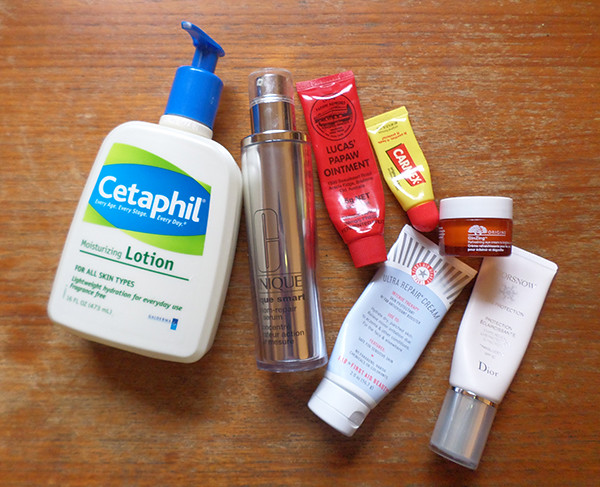A collection of skincare products is displayed on a worn wooden table with a bright brown hue. Prominently featured is a bottle of Cetaphil Moisturizing Lotion, with its distinct oval-square shape, blue squeezy top, and blue and green label. Adjacent to it is a sleek silver tube labeled Clinique Smart Custom-Repair Serum. A small red squeezy tube of Lucas’ Papaw Ointment stands next to it, alongside an even smaller yellow squeezy tube with a red top, identified as Carmex, marked by a red square with a white Carmex logo. Beneath these is a small orange jar with white writing and a matching white lid. Sitting near this jar is a white squeezy bottle from Dior. Completing the arrangement is a wider white squeezy bottle with blue accents, labeled Ultra Repair Cream by First Aid Beauty.